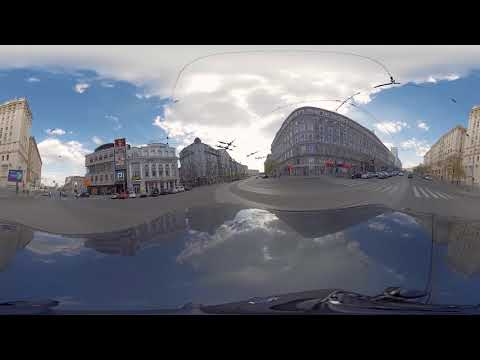The photograph captures an outdoor city street setting under a bright, sunny sky with scattered white clouds. Taken with a wide-angle lens from the viewpoint of someone driving a car, the image gives a slightly distorted, rounded perspective, emphasizing the curvature of the windshield and hood. The street is lined with various multi-story buildings exhibiting a classic, possibly European architecture, including a brown, tall building on the left, a gray three-story building to its right, and a four-story building further left. The main focal point is a sizable five-story building at a corner, presumed to be an apartment complex with stores at street level, flanked by a series of similar light sandstone buildings. The street is bustling with several cars, but no pedestrians are visible. A crosswalk stretches in front of these buildings, and hints of recent rain are evidenced by the damp streets, contributing to a relaxed atmosphere. The photograph, rectangular in shape with black headers and footers, intricately merges multiple images to create a wavy and dynamic visual effect, yet maintains a cohesive and picturesque cityscape scene.